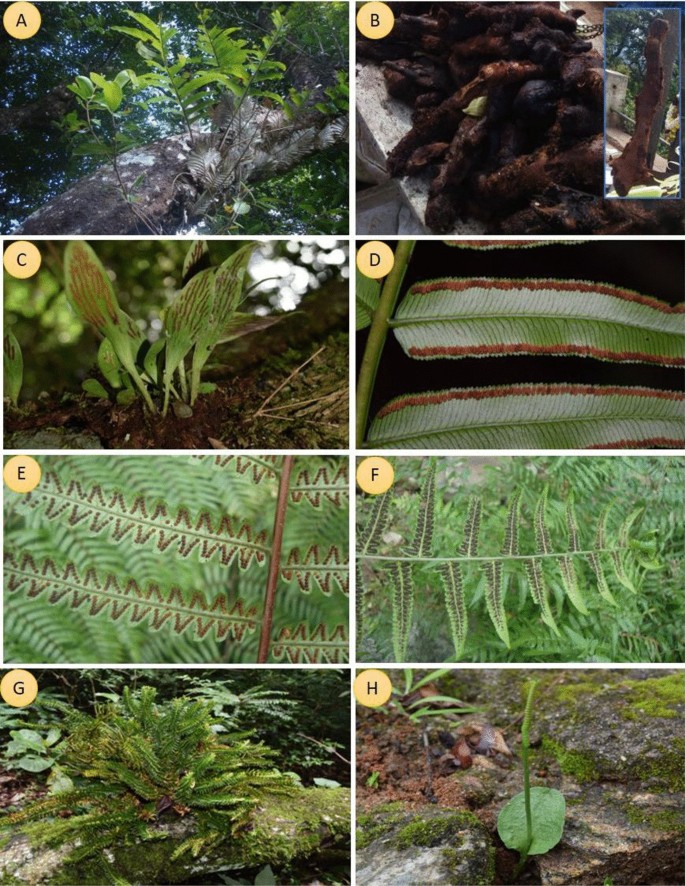A collage of eight color photographs (labeled A through H in tan circles) showcases different varieties of ferns, arranged in two columns of four rows. The images capture ferns at varying perspectives, from distant views to close-ups of the underside of fern leaves with visible spores. Notably, the photograph labeled B includes an inset that reveals a pile of brown, curled objects and an upright close-up, hinting at fern components. The series highlights the green and textured details of fern leaves, with a mixture of outdoor settings bathed in daylight. The photograph labeled D features a striking close-up of a white, waxy leaf with a brown border, while photo E presents a brown-stemmed leaf with brown and white zigzags. Overall, the collection provides a detailed, multi-angled exploration of fern structures and their natural habitats.